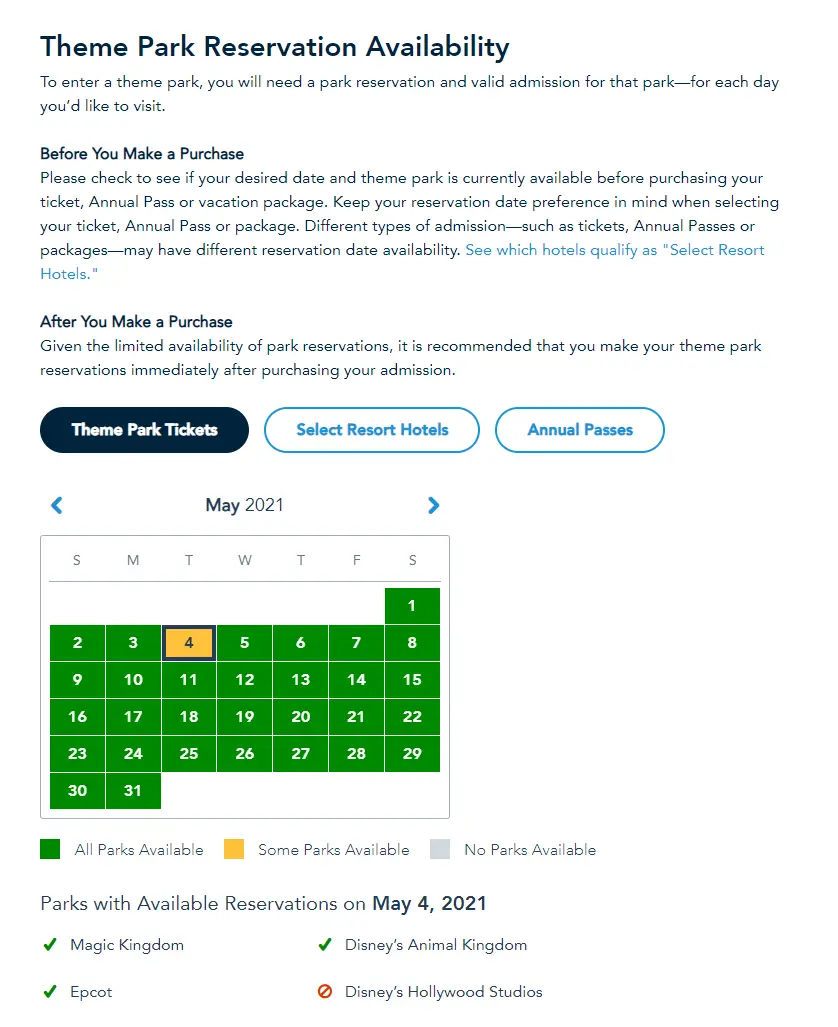In the provided image of a website, the background is predominantly white with dark text highlighting key information. At the top, the header reads "Theme Park Reservation Availability," with each word capitalized. 

Beneath this header, there's a brief explanation stating that visitors need both a park reservation and valid admission for each day they wish to enter a theme park. It advises individuals to check the availability of the desired date and theme park before purchasing tickets, annual passes, or vacation packages. Furthermore, it highlights that different types of admissions might have varying reservation date availabilities, and it suggests checking qualifying hotels for select resorts or accommodations.

Post-purchase instructions emphasize making theme park reservations immediately due to limited availability. 

The interface includes tabs, with the "Theme Park Admission" or "Theme Park Tickets" tab having a darker background with white text, whereas other tabs such as "Select Resort or Hotels" and "Annual Passes" have a light blue border against a white background.

A calendar interface is displayed showing May 2021, with navigation arrows on the left and right to move between months. The calendar dates have a green background with white numbers, except for the 4th, which stands out with a yellow background and a blue border.